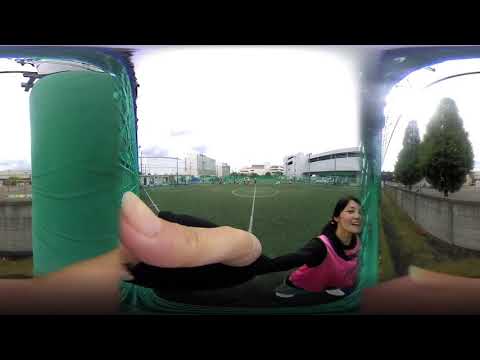The image captures a 360-degree view centered around a smiling woman with black hair, who is wearing a black long-sleeve shirt under a pink tank top that seems like a part of a uniform. She is seated and has her arm outstretched, likely holding the camera. Her sneakers are visible, and she is positioned slightly towards the bottom center of the frame. Surrounding her, there's a wide green field with white markings indicating a sports field—probably for soccer. 

In the background, various elements contribute to the rich details of the scene: several people are scattered across the field, a fence is visible to the left, and a small building, possibly a parking structure, can be seen to the right. Two trees stand towards the right side of the frame. The sky overhead is a mix of grey and white, adding to the outdoor, daytime setting which is well-lit by natural light. The image is bracketed by a black border at the top and bottom, providing additional structure to the 360-degree presentation, though this causes some visual warping typical of such panoramic images.